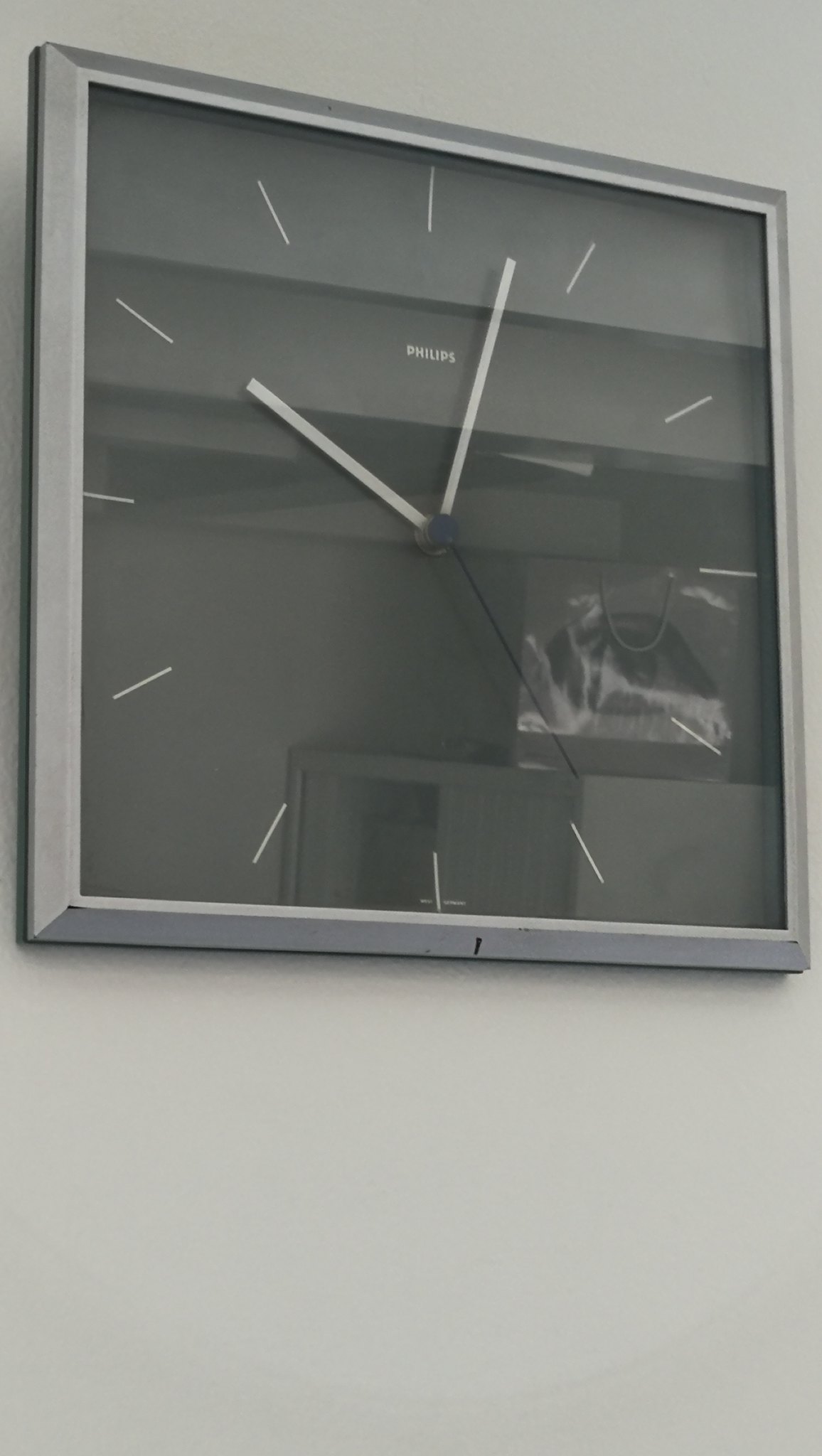This is a black and white photograph of a large, square wall clock, hanging on a white or off-white wall. The clock features a light-colored frame, possibly gray or silver, surrounding a shiny black clock face. Instead of numbers, the clock face displays small white lines to mark the hours. The word "Phillips" is written in white letters just above the clock's center. The clock has three hands: two white (minute and hour) and one black (second). The shiny surface of the clock reflects various objects from the room, including ceiling tiles, a picture of a turtle, and a column emerging from the top of a cabinet. Additionally, part of a gift bag with an eye design is visible in the reflection. The clock appears to show the time as approximately 10:03.